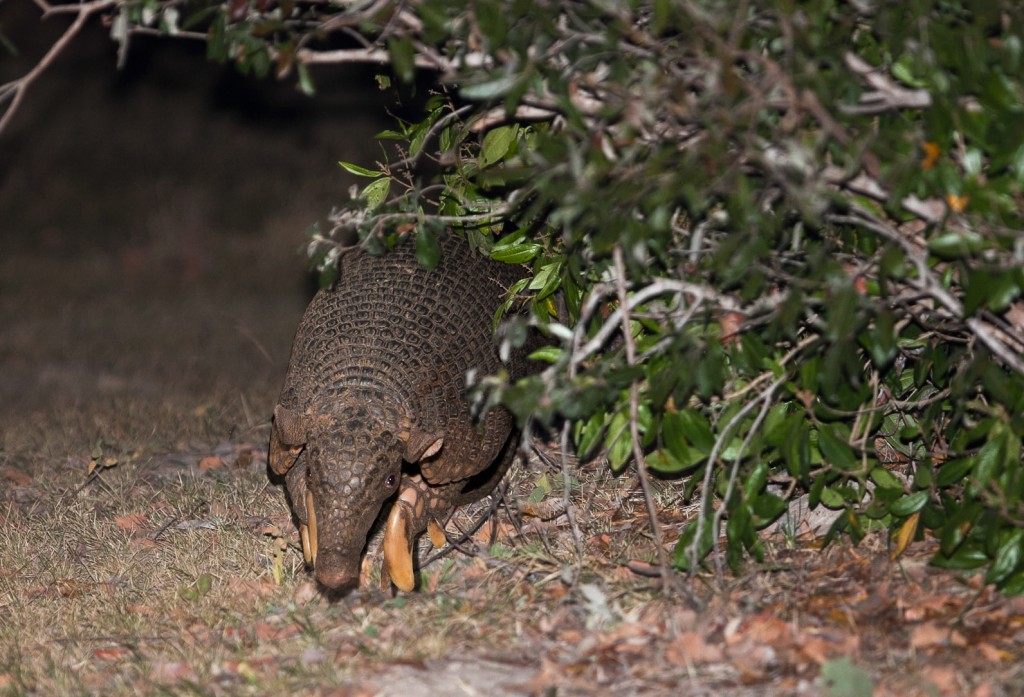In this captivating nocturnal photograph, a striking armadillo, bathed in the harsh glow of artificial light, reluctantly peeks out from the edge of some green yet somewhat faded brush. The scene is dominated by the armadillo's distinctive hard shell and its diminutive head, which is turned towards the camera, seemingly uncomfortable with the sudden brightness. This shy creature is caught mid-motion, showing only its head, two ears, front legs, and part of its armored body. The background is enveloped in darkness, hinting at a nighttime setting that the armadillo likely prefers. Surrounding the animal, the grass appears brown and dry, suggesting the photo was taken in late summer or early fall. Additionally, dried leaves are scattered across the ground, adding to the seasonal ambiance. The plant partially obscuring the armadillo adds an element of mystery to the image, enhancing the overall moodiness and reluctance of the solitary armadillo.